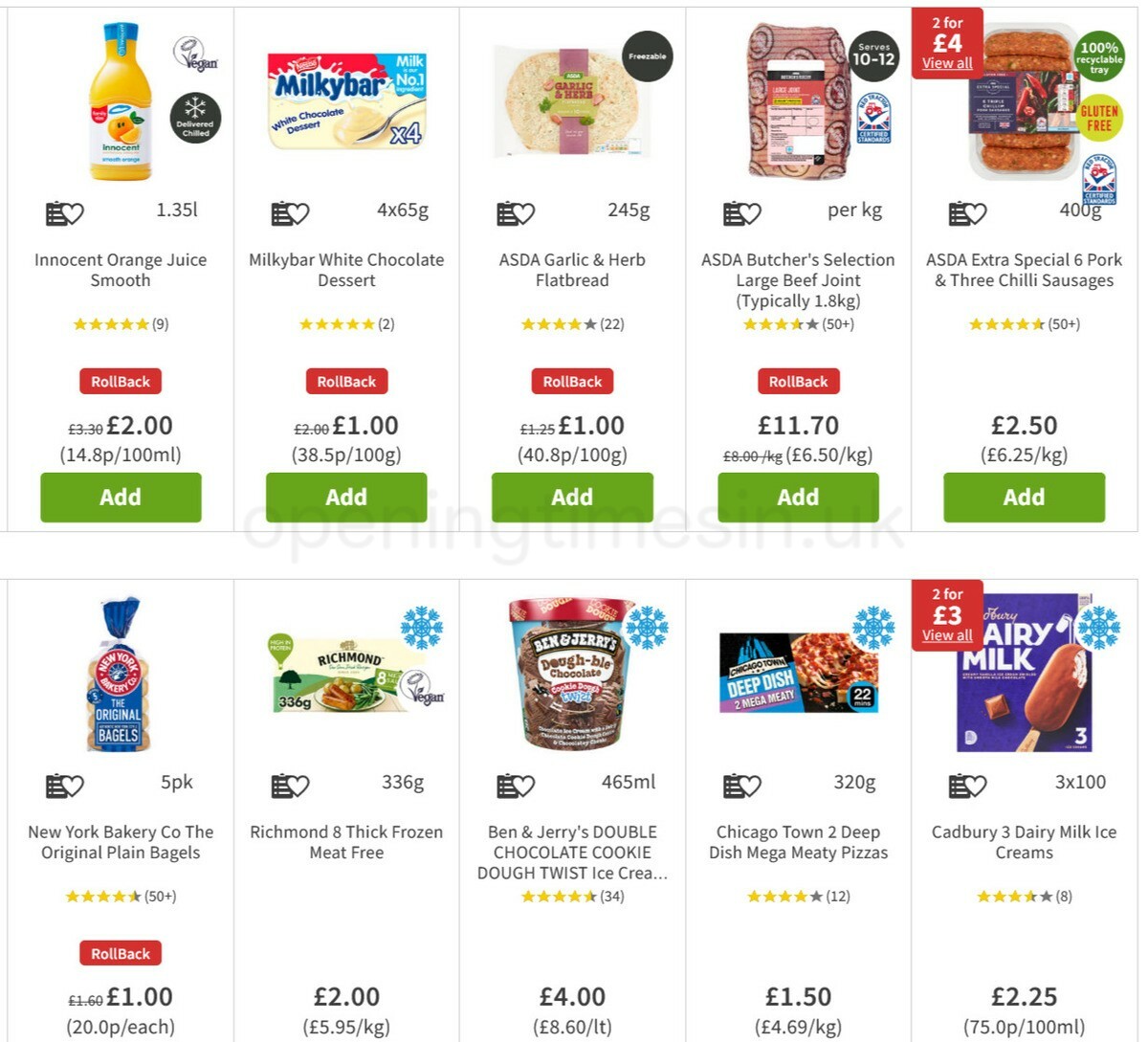Here's a detailed and cleaned-up caption for the given image:

---

The image showcases a UK-based online food ordering website featuring a selection of ten different food items arranged in two rows. Each item is displayed with a picture and its corresponding name. The first row includes the following items:

1. **Innocent Orange Juice Smooth**: Featuring an image of a bottle of orange juice.
2. **Milky Bar**: A white chocolate dessert depicted with a spoonful of the creamy dessert.
3. **Garlic and Herb Flatbread**: Displayed as a piece of seasoned flatbread.
4. **Large Beef Joint**: An image of a substantial cut of raw beef.
5. **Pork & Chili Sausages**: A package containing six pork sausages and three chili-flavored sausages.

The second row consists of:

1. **New York Bagels**: A visual of a bag of bagels.
2. **Richmond 8 Thick Frozen Meat Free Sausages**: A box containing eight thick meat-free frozen sausages.
3. **Ben & Jerry's Double Chocolate Cookie Dough Twist**: Illustrated by an image of the ice cream tub.
4. **Deep Dish Pizzas**: An image of prepared deep dish pizzas.
5. **Cadbury Dairy Milk Ice Cream**: A chocolate ice cream bar encased in a wrapper.

The pricing for half of these items is marked with the label "Roll Back," indicating discount prices.